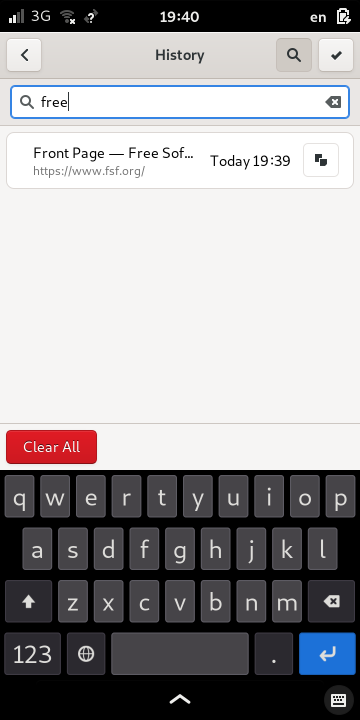A cell phone screenshot is displayed, depicting several user interface elements. At the top, there is a black rectangle containing the status indicators: on the left, the 3G reception bars and battery icon; the current time is centered; and on the right, a lowercase "¥" symbol followed by an icon. Immediately below this is a light gray rectangle. To the left of this is a back button, represented by a left arrow inside a box. At the center, in black text, it reads "History," and to the right, there are two buttons: a magnifying glass icon and a checkmark inside a button.

Below this section is a search bar, outlined in blue. It contains a magnifying glass icon to the left, followed by the text "free" with the vertical cursor line visible, and ends with a gray square with a white "X" inside on the right. Underneath the search bar is a white rectangle. On the left side in black text, it reads "Front page," followed by a double dash and "free sof..." indicating truncated text. Below this is a website address: "https://www.fsf.org/". On the right side of this section, centered in black text, it says "Today 19:39," next to a gray-outlined square containing two black boxes which are aligned such that the bottom right corner of one connects to the top left corner of the other.

The remaining space is mostly blank gray, save for a red "Clear all" button located on the lower left. At the very bottom is a keyboard interface.